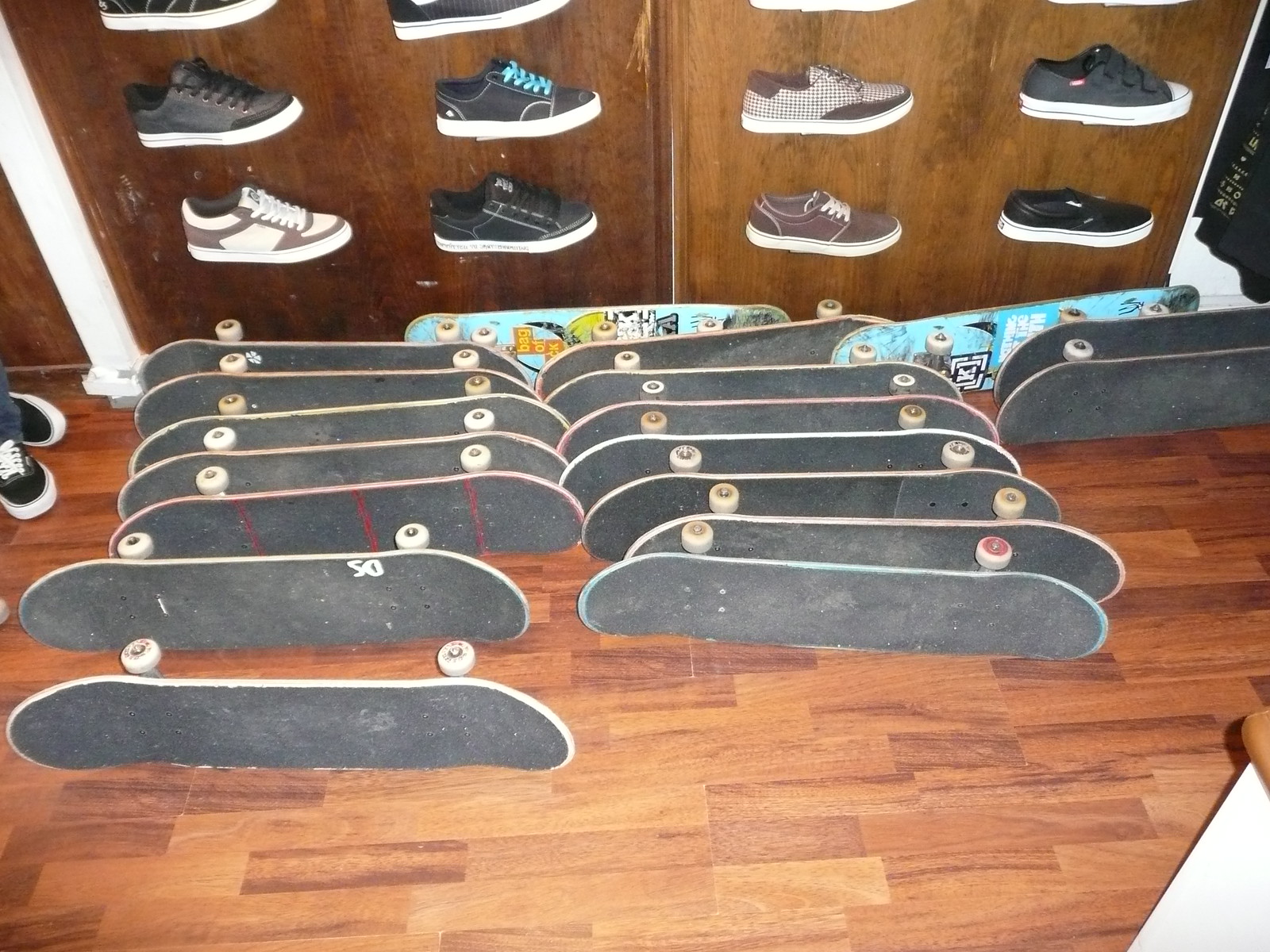The image captures a storefront display featuring a lineup of skateboards and an array of Vans shoes. The foreground showcases multiple skateboards laid side-by-side on a wood parquet floor, predominantly exhibiting their black grip tape and equipped with white wheels. These skateboards mostly show signs of use and, amongst them, a few feature a blue print design. The background displays a wood-paneled wall adorned with small shelves, each presenting a single Vans shoe. The shoes come in various colors and patterns, including a mix of black, white, tan, brown, and even a houndstooth design. On the left side of the wall, a white and tan shoe stands out, alongside multiple black shoes, with one sporting blue laces. The lighting appears to be from a flash, accentuating the textured details and creating a crisp, detailed view of both the skateboards and the shoes.